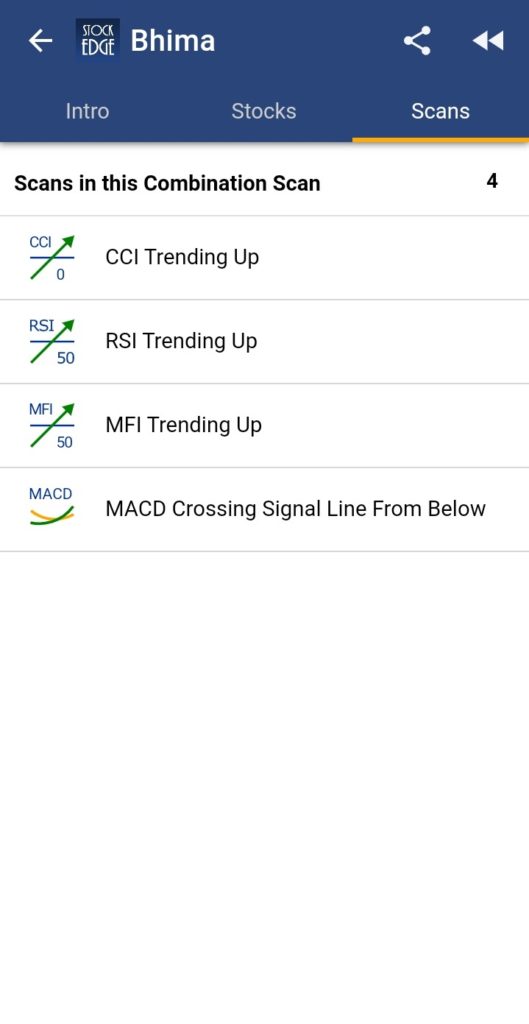This is an elongated screenshot of the BEMA Stock Edge app interface. At the top is a blue ribbon with white text. On the left side of the ribbon, there is an arrow pointing left, followed by the text "Stock Edge." To the right of that, it reads "BEMA (B-H-I-M-A)." Adjacent to the text are a play symbol and a linking symbol. Below this, still within the blue ribbon, the words "Intro," "Stocks," and "Scans" are displayed in white font.

The main section of the image has a white background with bold black text that reads "Scans in this combination: Scan." Beneath this header, stock indicators are listed: "CCI Trending Up," "RSI," "MFI Trending Up," and "MACO Crossing Signal Line from Below." It appears to be a stock alert app summarizing trends in specified stocks that the user is monitoring.

The screenshot is noticeably stretched, suggesting it was resized larger by the user, which has distorted the image.